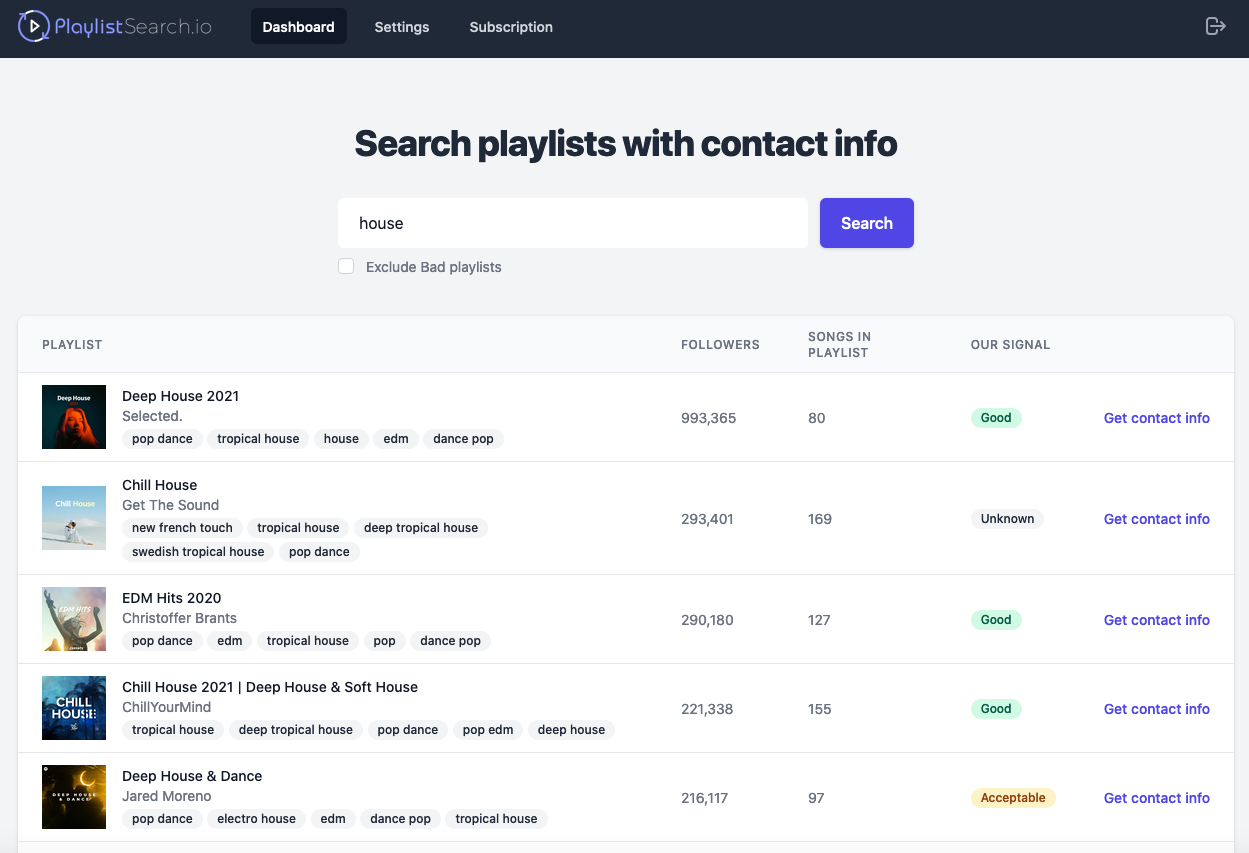This image displays a screenshot of the Playlist Search.io website. The top bar of the interface is black with three menu options: "Dashboard," "Settings," and "Subscription," all written in white, indicating the current focus is on the "Dashboard."

In the main section of the webpage, there is a prominent header that reads "Search playlists with contact info." Below this header is a search bar pre-filled with the word "house" and an adjacent search button encased in a bluish-purplish box. There is a tick box option available to exclude bad playlists from the search results.

Five different playlist options are presented on the page. The first playlist, titled "Deep House 2021," is selected and tagged with "Pop Dance," "Tropical House," "House," "EDM," and "Dance Pop." It boasts 993,365 followers and contains 80 songs. The status indicator shows that the signal is good. There is also a conspicuous blue button labeled "Get Contact Info."

The second playlist is called "Chill House" and includes tags such as "New French Touch," "Tropical House," "Deep Tropical House," "Swedish Tropical House," and "Pop Dance." This playlist has garnered 293,401 followers and comprises 169 songs. The signal status is marked as unknown, and it also features a blue button to retrieve contact information.

The third playlist listed is "EDM Hits 2020" created by Christopher Brands. Its tags include "Pop Dance," "EDM," "Tropical House," and "Pop." This playlist has 290,180 followers and contains 127 songs. The signal indicator reads good, and similar to the other listings, there is a blue button for obtaining contact information.